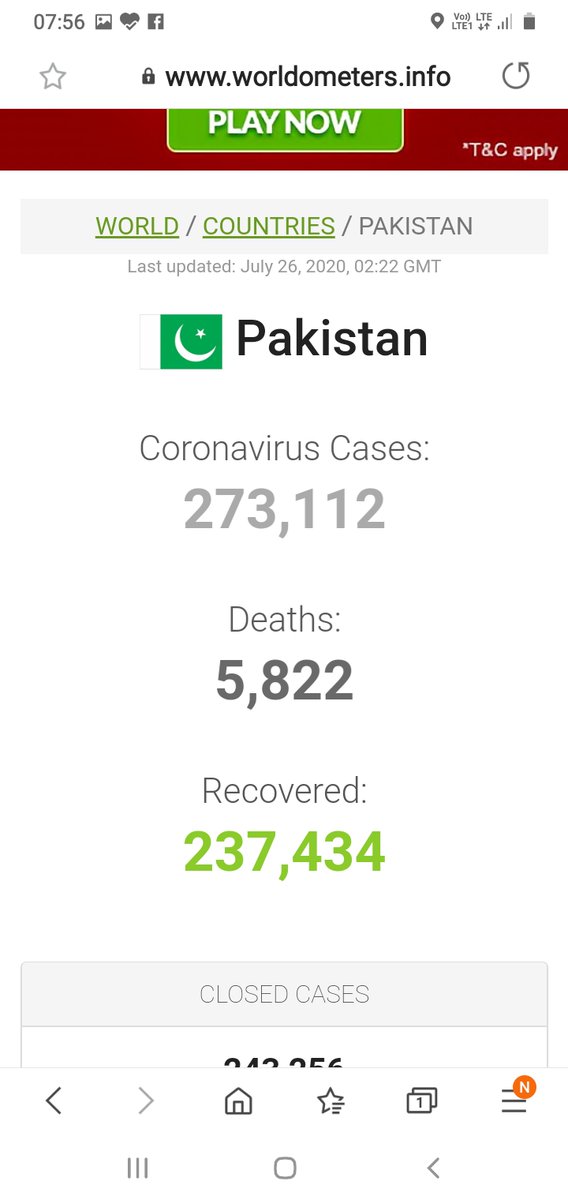Detailed Caption: 
The image displays a screenshot of a webpage on a smartphone, evidenced by the nearly full battery icon at the top right corner. At the top left, there is the Facebook logo. Below the address bar, which reads "www.worldometers.info," is a green rectangle. The page is headlined with "Country," followed by "Pakistan," and the current date of the last update, "July 26, 2020." 

The page details the coronavirus statistics for Pakistan, highlighting the number of cases: 273,112, deaths: 5,822, and recovered: 237,434. A pair of navigation arrows, one grey pointing to the right and one pointing to the left, suggests the availability of more data. 

Accompanied by the flags and common symbols like building icons and a hamburger menu, this detailed breakdown offers a concise snapshot of the COVID-19 situation in Pakistan as per the specified date.